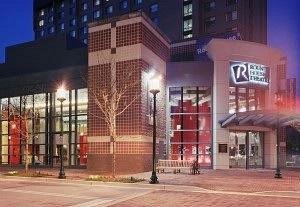This image captures a nighttime street corner scene featuring a modern retail storefront. The primary building, which appears to be a store, displays a prominent "R" logo in the upper right, set in a slightly tilted square that is wider at the top. The store façade is characterized by large windows with rectangular panes, offering a glimpse of red and white interiors, likely illuminated by the ambient lighting from the glass awning above the entrance. A white park bench is positioned outside, adding to the urban streetscape. The sidewalk, along with various walkways, is paved with bricks in different hues, contributing to a visually appealing environment.

Flanking this storefront is a larger, possibly residential building in the background, having numerous lit windows that suggest apartment units. The sky varies from a deep blue in the upper left to a purplish hue in the upper right, which may result from the lighting of the main building. Situated on a clean, quiet street devoid of pedestrians or vehicles, the scene includes distinctive antique-looking streetlights that illuminate the area. The storefront sits at an apparent intersection marked by a stop bar, and the lack of activity hints at a serene urban nightscape. The overall setting suggests a newly developed area, possibly in a city with historical influences, exemplified by the brick architecture and classic streetlamps.